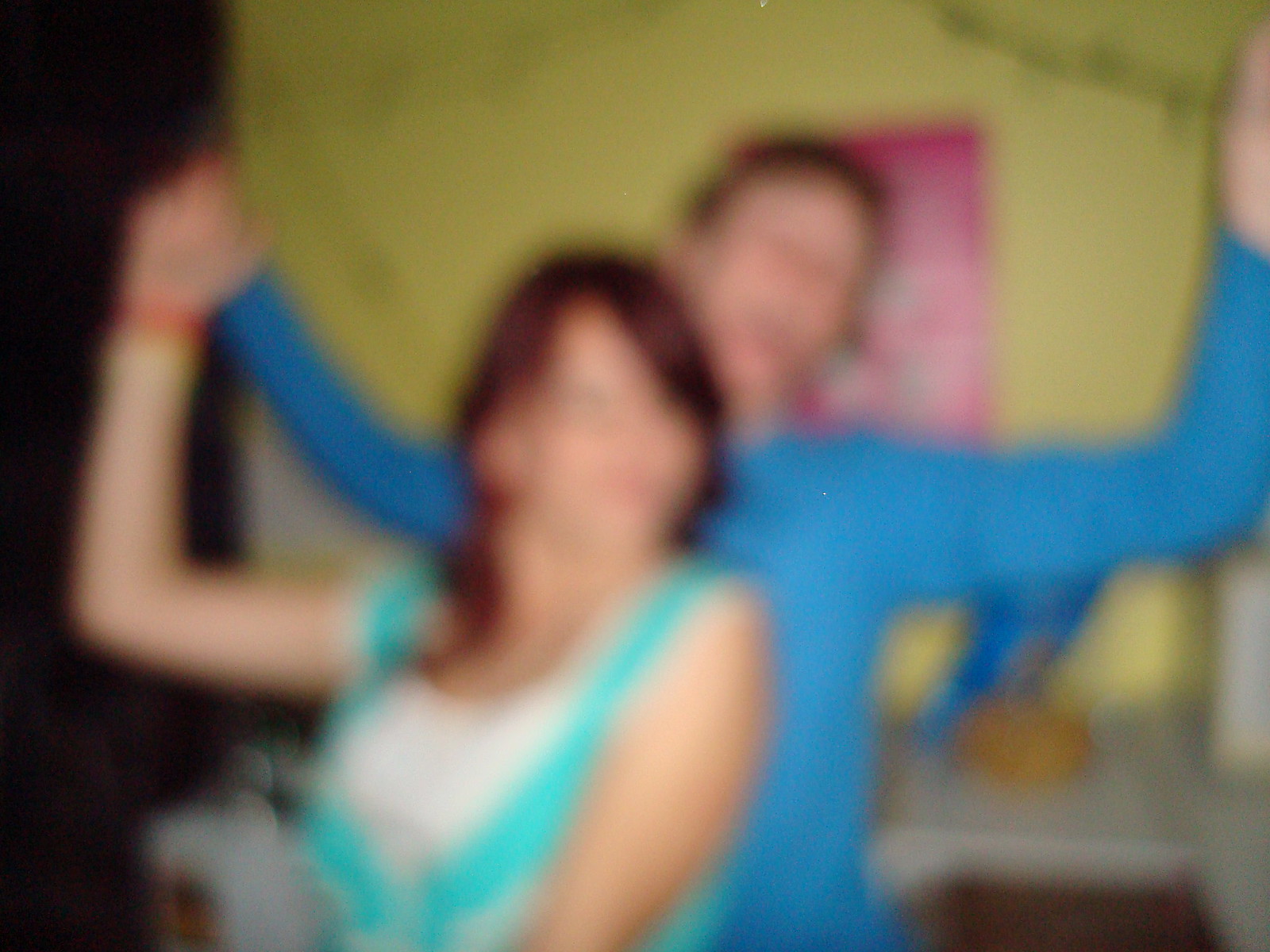This photograph captures a lively moment between two people, seemingly taken at a party. The image is slightly out-of-focus, creating a sense of motion and excitement. In the background, there is a green wall adorned with a pink poster, while a gray countertop below holds a blue bag and some brown items, adding context to the setting.

In the foreground, a young man is seen with his arms raised in the air, his head tilted back, and his mouth open in a joyful expression. He has brown hair and is wearing a bright sky-blue shirt, which adds a vibrant contrast to the scene. 

In front of him stands a woman whose right arm is also raised, as if matching his enthusiasm. She wears a white top accented with aquamarine on its edges and has a wristband on her right wrist. Her reddish-brown hair is swept back, complementing the overall dynamic and festive atmosphere captured in the photograph.